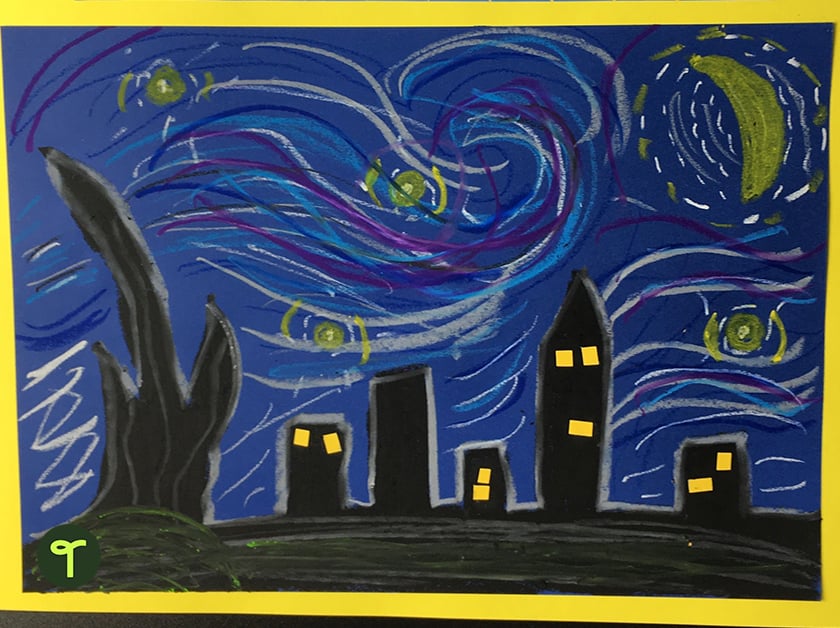The image depicts a vibrant night scene reminiscent of "Starry Night" by Vincent van Gogh, with the sky dominated by dramatic swirls of light blue, dark purple, white, and black, creating a dynamic impression of wind and movement. The moon, appearing almost like a yellow banana, shines brightly in the upper right corner, surrounded by numerous yellow stars or possibly fireflies that add to the whimsical feel. Framed by a yellow border, the scene has a blue background filled with these swirling patterns.

Below the tumultuous sky lies a stark, black terrain featuring five distinct black buildings of varying shapes and sizes. Most structures sport small yellow squares, indicating illuminated windows, except for one windowless building. One of the buildings has a pointed roof, diverging from the flat roofs of the others. To the left of these buildings stands a dark, tree-like stump or bush, adding an element of nature to the urban depiction. The whole composition gives a sense of a child's imaginative interpretation, possibly created with chalk or crayon-like textures on dark paper.